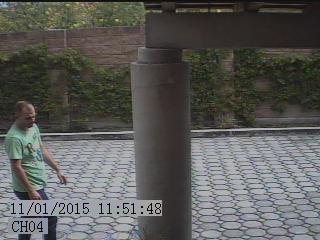In this photorealistic image captured from a video camera, we see an outdoor path composed of interlocking circular gray tiles. Dominating the center is a large stone or concrete pillar that extends upwards and out of the frame, suggesting it supports a structure off to the right, possibly a bridge. On the left side of the image stands a man with dark, slightly balding hair, dressed in a green t-shirt with red, yellow, and blue writing, and dark blue jeans. He appears to be walking leftward, his arms extended slightly in front of him, and looking down and to the right. The background features a brown stone fence adorned with green ivy and climbing vines. Additionally, some trees are visible behind the wall. The bottom left corner of the image contains two gray bars, the top one displaying the timestamp "11-01-2015 11:51:48", and the one below marked with “CH04” in black writing, indicating Channel 4 video footage.